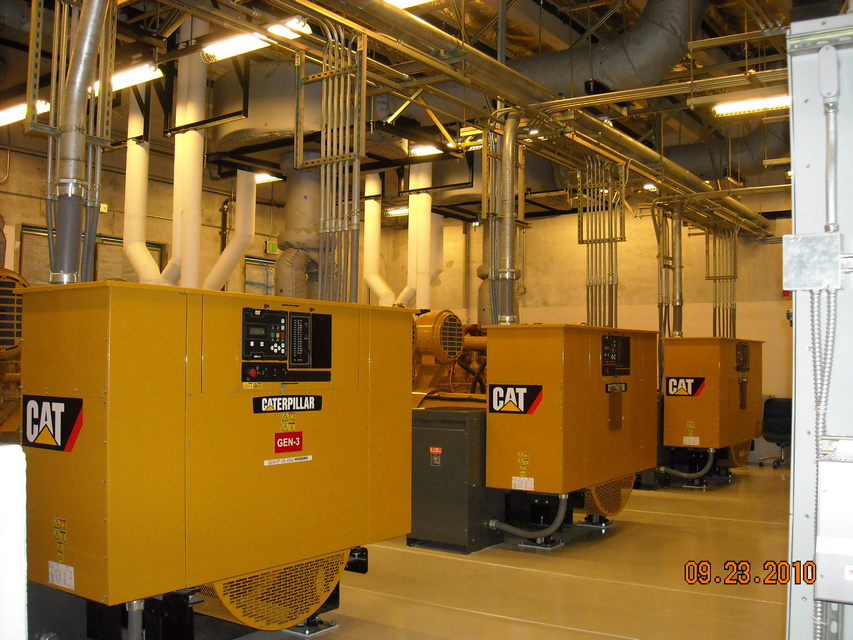The photograph, dated 09-23-2010, shows an industrial generator room possibly within a factory or storage facility. The prominent feature is three large Caterpillar-branded machines in a bright yellow or mustard color which are labeled as Gen-3 Cat. These machines have black keypads and a workspace on the front, along with detailed data boards and areas with venting grates at the bottom. A complex network of pipes, ducts, and silver metal venting tubes connects the machines to the ceiling, creating an intricate, crisscrossing web that obscures the ceiling itself. The floor appears to be made of laminate. An orange timestamp marks the bottom right corner of the image, reminiscent of old digital cameras. Industrial lighting illuminates the scene, highlighting the technical intricacies of the equipment.